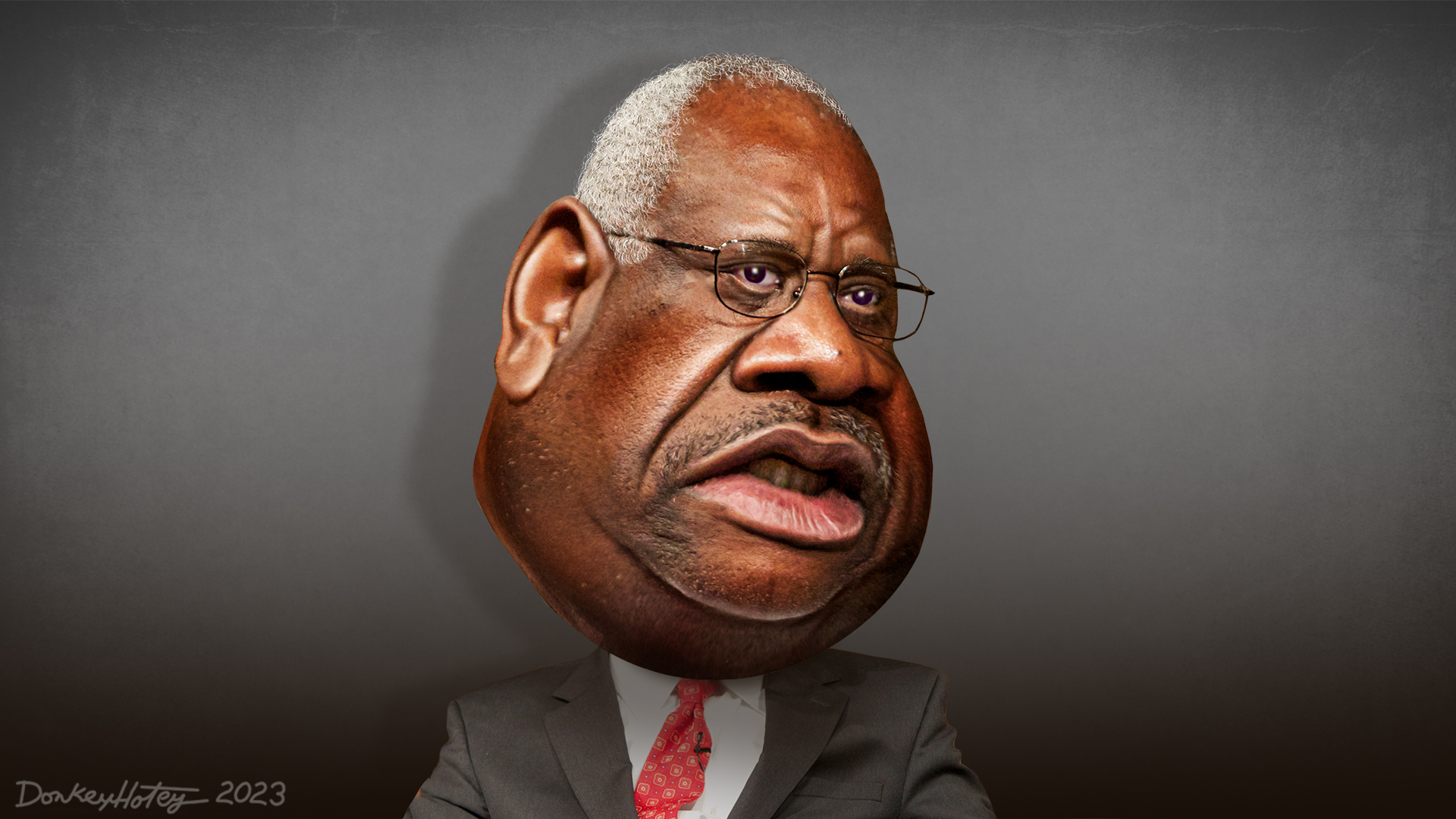The image is a heavily edited photograph featuring a person with an exaggerated, caricatured head. The background of the image is a gradient of gray, lightening towards the center and darkening towards the edges until it turns black. In the bottom left corner, there is semi-transparent white text that reads "Don Quixote 23." The person is visible from the chest up, wearing a gray business suit, a white button-up shirt, and a red tie with white dots, which has a small lapel microphone attached. The person's head is disproportionately large, pear-shaped, and made to appear much bigger than their body, creating a caricature effect. They have gray hair, a thin mustache, eyeglasses, chubby cheeks, and they're looking towards the right. The photograph appears to be digitally manipulated, possibly using software like Adobe Photoshop.